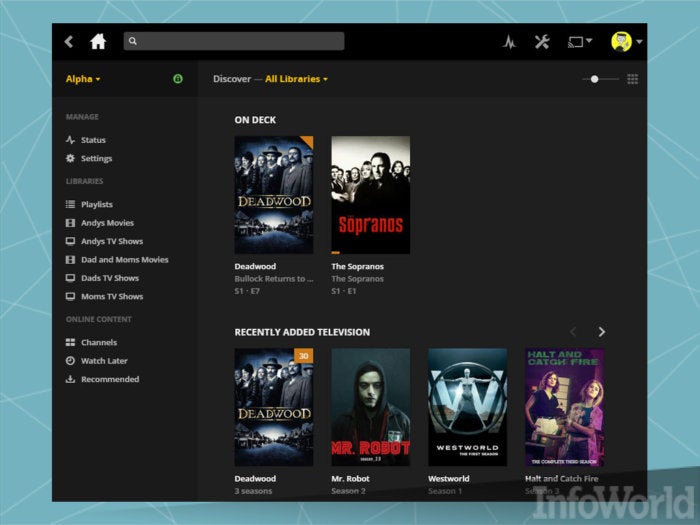The image features a digital interface from a page titled "Info World." The entire background is a teal color interspersed with subtle white lines that traverse the backdrop. Positioned in the lower-right corner, the semi-transparent text "Info World" stands out, blending into the colorful scenery.

At the top of the image, a small house icon and a search button are prominently displayed. Scattered around this section are various icons, including a profile picture resembling a cartoon character, along with some tool icons and a drop-down menu.

Below, the heading "Discover" is highlighted in yellow, next to the text "All Libraries." Further down, the section labeled "On Deck" features the TV shows *Deadwood* and *The Sopranos*. Continuing downward, a segment titled "Recently Added Television" showcases titles such as *Deadwood*, *Mr. Robot*, *Westworld*, and *Halt and Catch Fire*.

On the left side of the screen, the word "Alpha" can be seen in yellow, accompanied by a drop-down menu. Below this, the navigation options include "Manage," "Status," "Settings," "Libraries," and "Online Content." The overall layout is organized and filled with icons and text that help users navigate through different sections of the interface seamlessly.